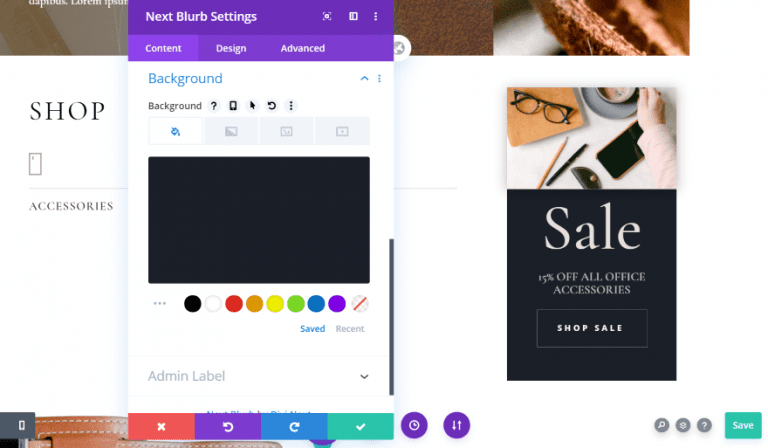The image depicts a website interface featuring an overlay that appears to be part of its functionality. The background of the website includes a prominent top photo banner with shades of brown and gray on the left, transitioning to an indistinguishable picture on the right. Below this banner, on the right side, there is an image of a desk setup with various objects including glasses, pens, a phone, a warm beverage, and a person's hand, suggesting a workspace scene.

Further down, a black section with white text announces a promotional offer: "15% off all office accessories." Beneath this announcement lies a "Shop Sale" button with white text and a grayish border, inviting users to explore the offer.

Central to the image is an overlay dialogue box with a purple header stating "Next Blurb Settings" in white text. The header also contains icons for expanding the dialogue box, possibly including a menu icon and other function-related symbols. The dialogue box features three main tabs—Content, Design, and Advanced—displayed in a lighter purple when selected (Content is currently selected).

Within the dialogue box, the term "Background" is highlighted in blue text with a drop-down arrow and a three-dot vertical menu beside it. Below this heading, the term "Background" appears again with several control icons including a question mark, a rectangle, an arrow, a refresh button, and three dots. A pink paint can icon is shown as selected, paired with a white background and blue text, while adjacent grayed-out icons depict options for a picture, a chart, and a video (a rectangle with a triangle).

Following this, there is a solid black box and below it, three-dot menu indicators on the left alongside a series of color selection icons displayed as round buttons. These colors include black, white, red, orange, yellow, green, blue, purple, and a transparent option with a diagonal red line. The term "Saved" is displayed in blue text on the left, indicating it is the current selection, with "Recent" grayed out beside it.

At the bottom of the dialogue box, the term "Admin Label" is presented with a down arrow, followed by partially visible blue text and a series of action icons positioned below. These icons include a red background with a white X, a blue-purple background with a back arrow, a blue background with a forward arrow, and a green background with a white checkmark.

This detailed description captures the structured layers and various elements of the website interface and its overlay, giving a clear visualization of the design and functional components presented.